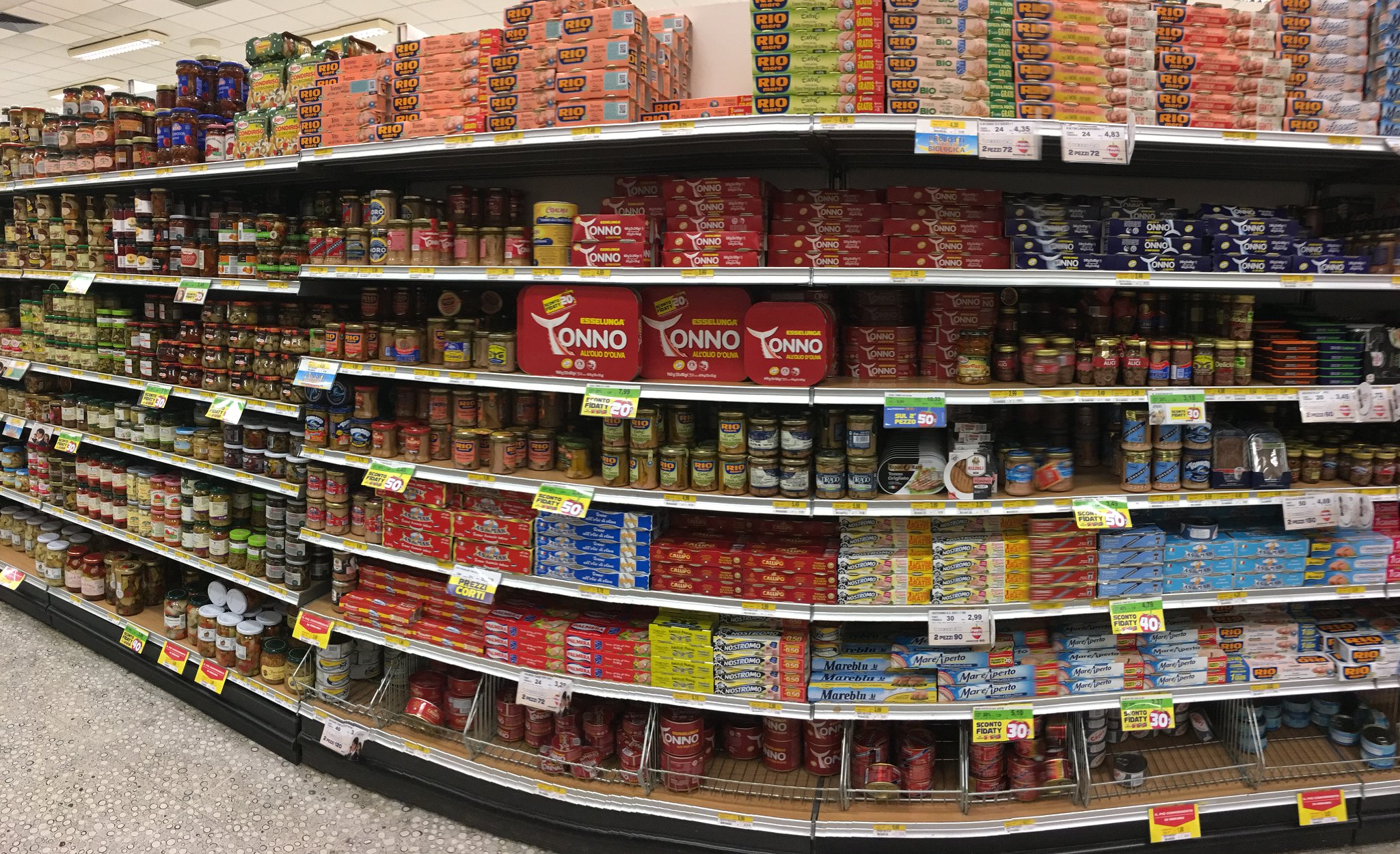This photograph captures a well-organized, rounded shelving display in a store, featuring six distinct levels of neatly arranged products. The top shelf is densely stacked with various boxes. On the second and third shelves, boxes are piled to the right while an assortment of cans and jars occupy the left side. The fourth shelf is dedicated entirely to an array of cans and bottles. Similarly, the fifth shelf mirrors the structure of the second and third, with boxes to the right and jars and cans to the left. The bottommost shelf is divided by wire separators, each compartment filled with an assortment of cans. Bright yellow signs with red squares are prominently attached to the front of each shelf, possibly indicating promotions or pricing.